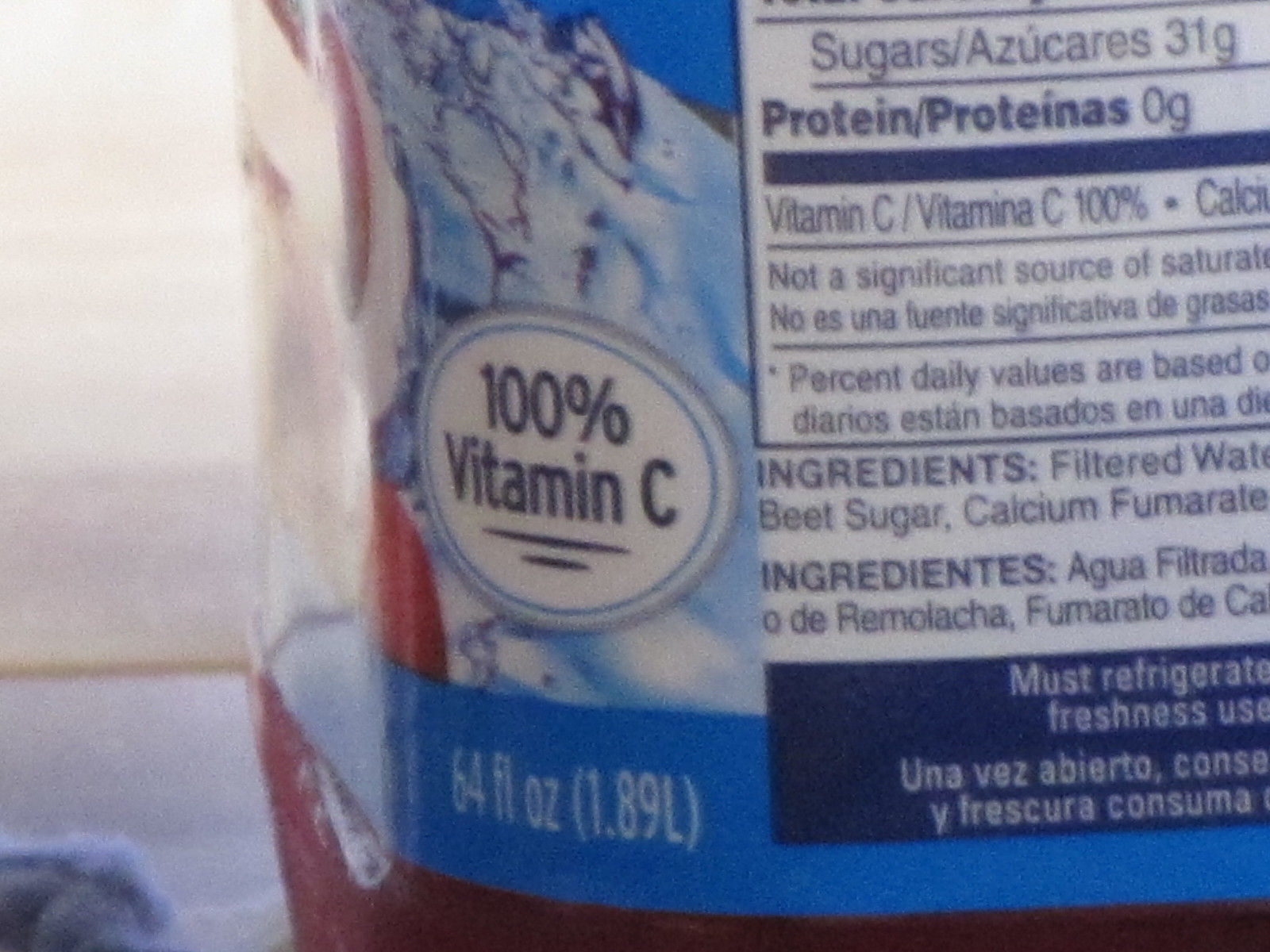Close-up of a Cranberry Juice Bottle’s Back Label

This detailed close-up image captures the back label of a 64 fluid-ounce cranberry juice bottle. The prominent brand logo highlights "100% Vitamin C," set against a background graphic featuring a snowy mountaintop. Due to the zoomed-in nature of the photograph, the front and sides of the bottle are not visible. The partially shown nutrition facts chart reveals information up to the sugar content, followed by entries for protein, vitamin C, and calcium. Additionally, a segment of the ingredient list is visible, though incomplete due to the tight framing of the shot.